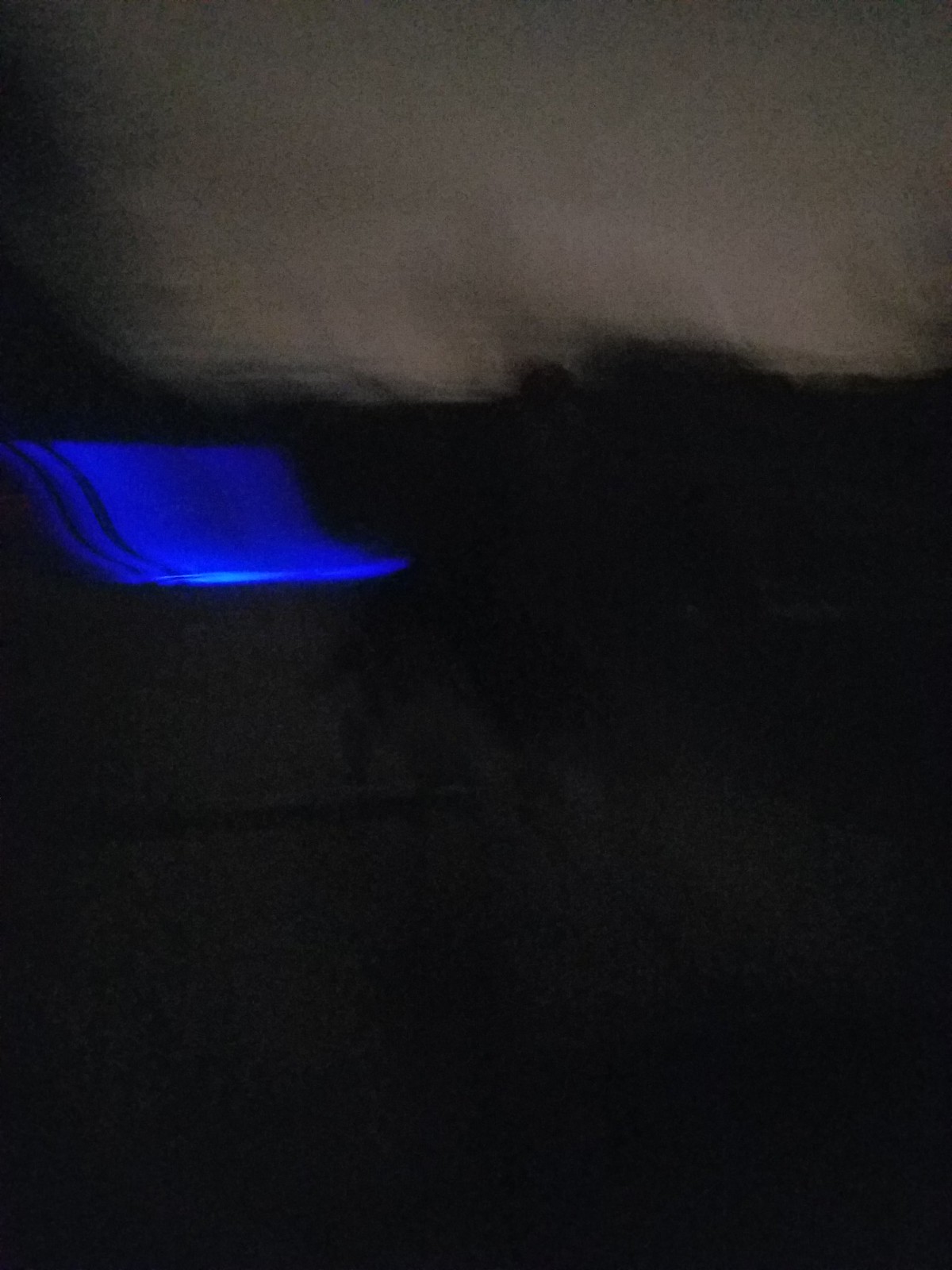The image portrays a striking contrast between brightness and darkness. The upper section is dominated by a bright, white area, while the lower part is enveloped in deep black tones. On the left-hand side, there is a distinct, blurry swirl of blue light, suggesting dynamic movement. This blue hue resembles the glow of an LED light, its fuzzy edges contributing to the overall out-of-focus impression of the scene. The background seems to reflect a gray sky, void of any discernible shapes or forms, emphasizing the swirling blue light's kinetic energy against a stark color palette.